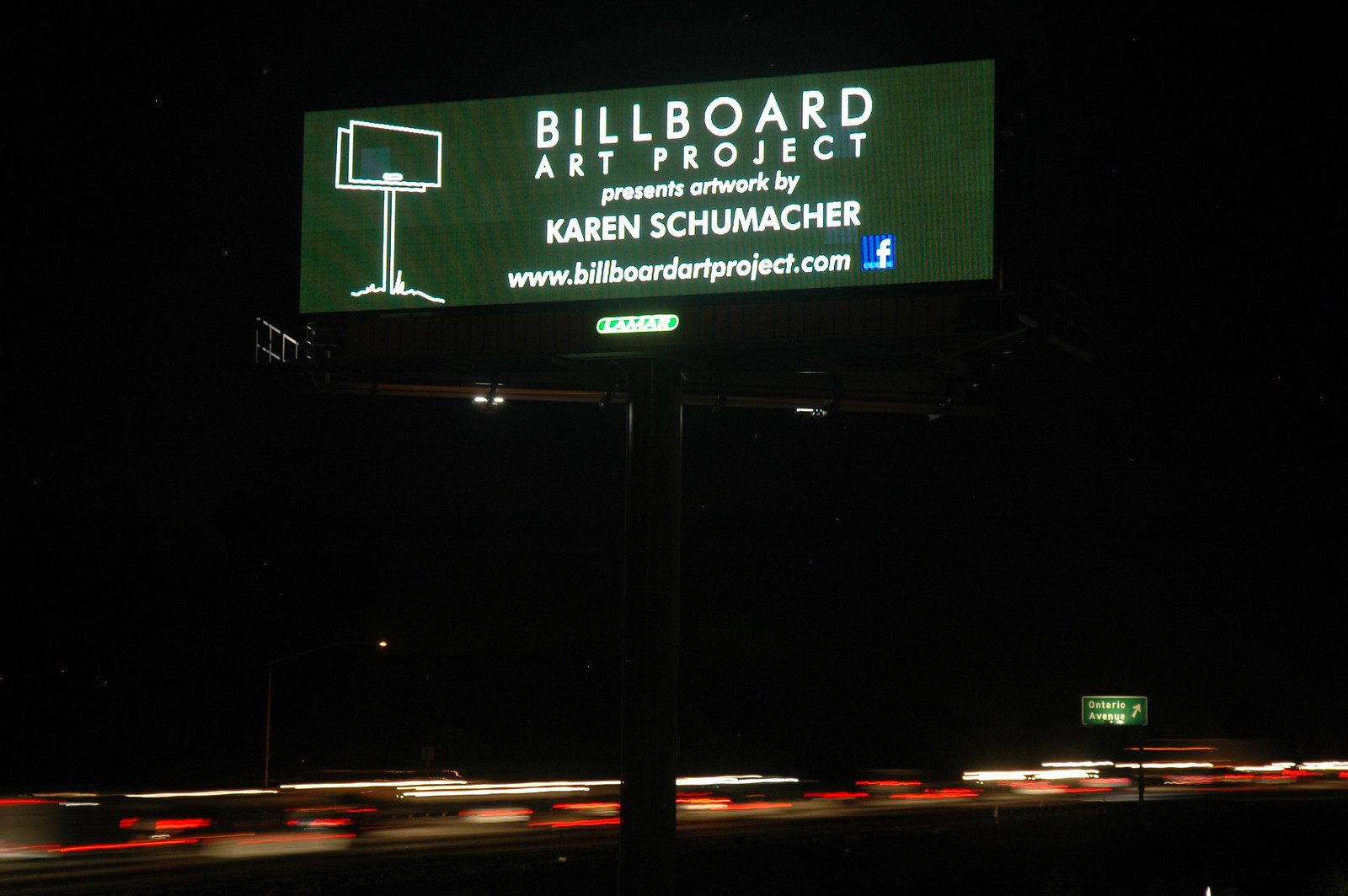A nighttime photograph captures a large billboard positioned along a busy road or motorway. The background is predominantly black, filled with the darkness of the night sky. The billboard, prominently illuminated, features a dark green backdrop. On the left side of the billboard, there is a white line drawing of a billboard standing amid grassy terrain. Bold capital letters at the top of the billboard spell out "Billboard Art Project." Below this, it reads, “Presents artwork by Karen Schumacher,” along with the website address "www.billboardartproject.com," which is accompanied by a Facebook icon. The billboard is produced by Lamar, with their elongated oval logo placed at the bottom.

The foreground features a road where cars are seen as streaks of light due to a long exposure setting, making their red taillights and white headlights appear as blurred lines, denoting their movement in opposite directions. To the right of the scene, a road sign directs drivers towards Ontario Avenue. The clarity of the billboard contrasts sharply with the dynamic, blurred motion of the cars, creating a captivating interplay between the stillness of the advertising medium and the bustling nighttime traffic.